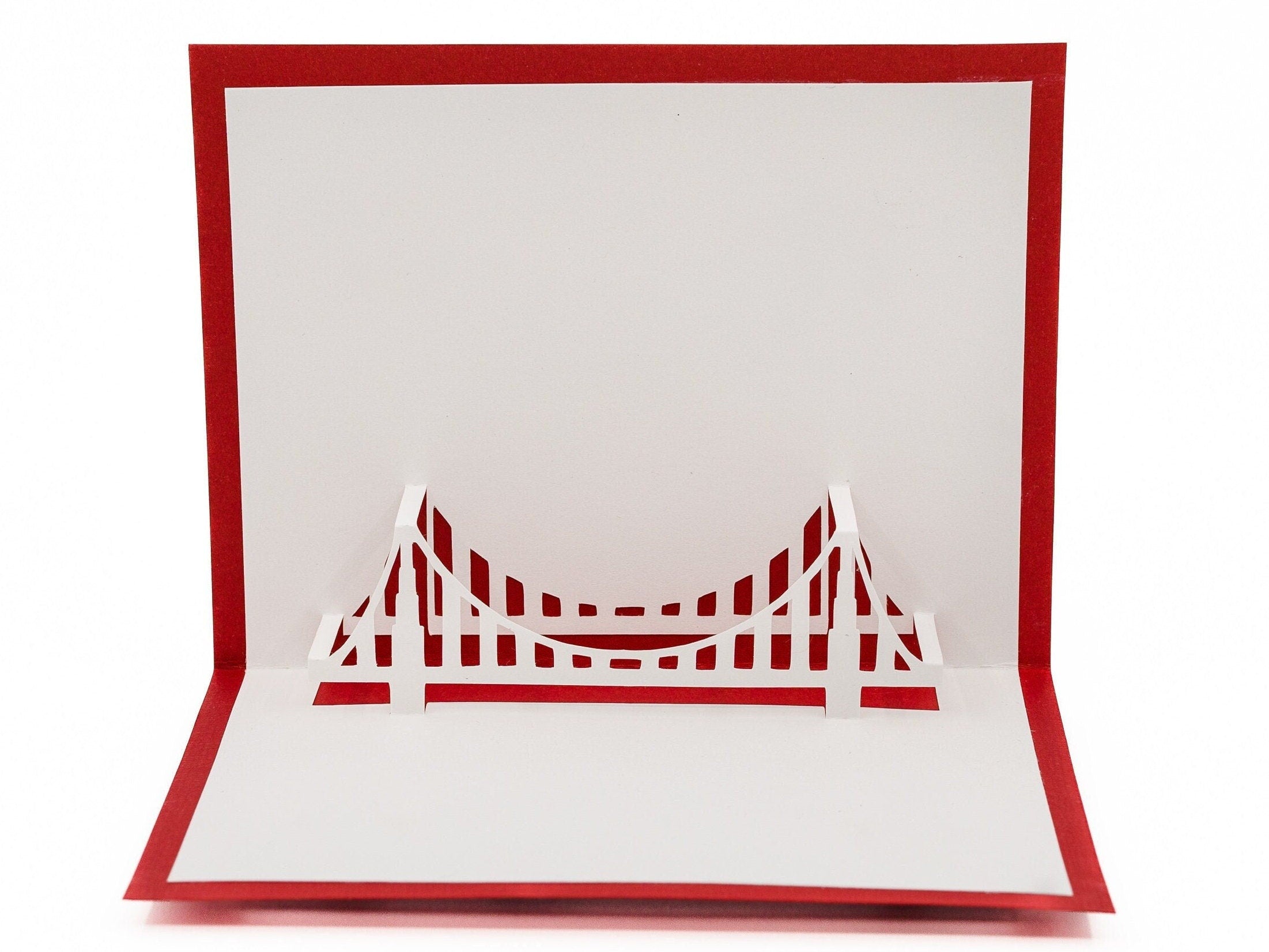The image depicts a meticulously crafted three-dimensional pop-up scene created from paper. A white sheet of paper with intricate cuts is layered over a red background paper, creating a striking contrast. When the white paper is folded and opened, it reveals a skillfully designed suspension bridge with posts on either side and an arch in the middle. The red background shows through the cutouts, enhancing the details of the bridge structure and adding depth to the paper art. There is no text or descriptions on the paper, allowing the detailed paper-cut art to stand out. While the specific bridge's identity remains ambiguous, it evokes the iconic structures of well-known suspension bridges like those in San Francisco or New York.